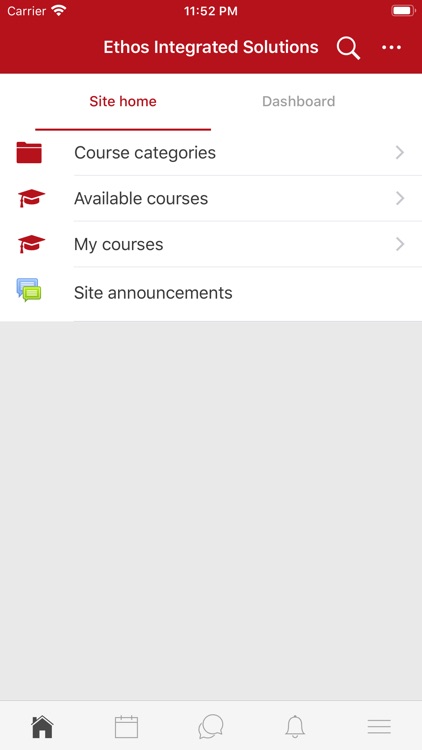The image showcases the dashboard of "Ethos Integrated Solutions," with the title prominently displayed in a red bar at the top. The status bar indicates a strong network connection with full signal strength and a battery at 100%, shown at 11:52 PM. 

Below the status bar, a navigation area includes a search bar accompanied by three vertical dots (likely for additional options). Directly beneath, two primary menu choices are visible: "Site Home" and "Dashboard," with "Site Home" currently highlighted in red, indicating its active status.

Further down, there's a navigational menu featuring expandable sections such as "Course Categories," with a blue-red box icon, "Available Courses" marked by a graduation cap icon, and "My Courses," also represented with a graduation cap icon. "Course Categories" and "Available Courses" are configured as drop-down menus.

The dashboard includes a section titled "Site Announcements," identified by two computer icons—one blue and one green. However, this section is notably large and devoid of any content or announcements, exemplifying its empty state.

The default home screen is indicated by a highlighted gray box, suggesting that all initial navigations will start from this point. This area is where users would write or post announcements, as implied by the layout and highlighted elements.